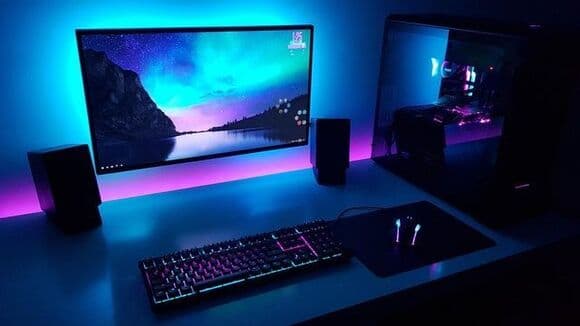The image depicts a darkly-lit desktop gaming setup, accented by vibrant LED lights. The main feature is a large, wall-mounted monitor displaying a nature scene at night, complete with an aurora borealis over a serene lake flanked by mountains and trees. Beneath the monitor, a keyboard and a mouse sit on a computer desk, both illuminated by pink and teal blue LED lights that emphasize the relaxed and calming atmosphere of the room. The desk is flanked by two desktop speakers on either side of the monitor. The LED lights, primarily pink and teal blue, illuminate the space from behind the desk and monitor, providing a soft, ambient glow. Despite the absence of a visible chair, the setup suggests a cozy and quiet workspace. To the far right, the dark room hints at various indistinct objects, possibly a computer tower and a cabinet, which merge into the shadows.